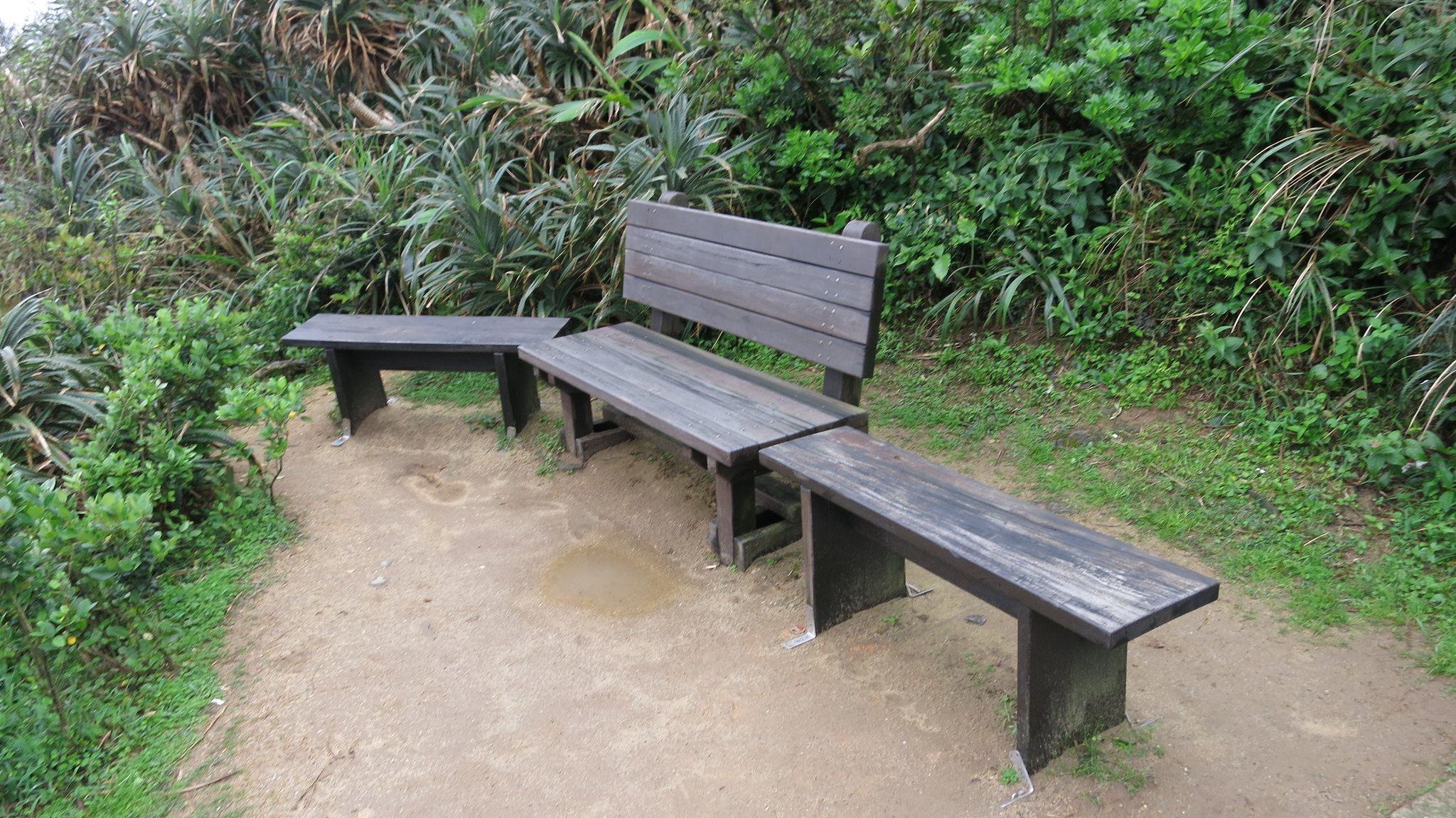The image depicts a serene corner in a lush tropical garden, characterized by dense, thick foliage with small palm trees and various other green plants. The ground is primarily damp, sandy soil with scattered patches of grass. This outdoor space features a trio of wooden benches arranged closely together. On the left, there is a simple, dark-colored wooden bench without armrests or a backrest, angled to lean against a central park-style bench. This central bench, also wooden, has a sturdy frame and a supportive backrest. To its right, another long, flat bench with rectangular legs is positioned alongside the main bench. The setting evokes a peaceful, relaxing atmosphere, likely near a beach, where one could sit and gaze at an imagined stunning ocean view, surrounded by the vibrant, tropical greenery.